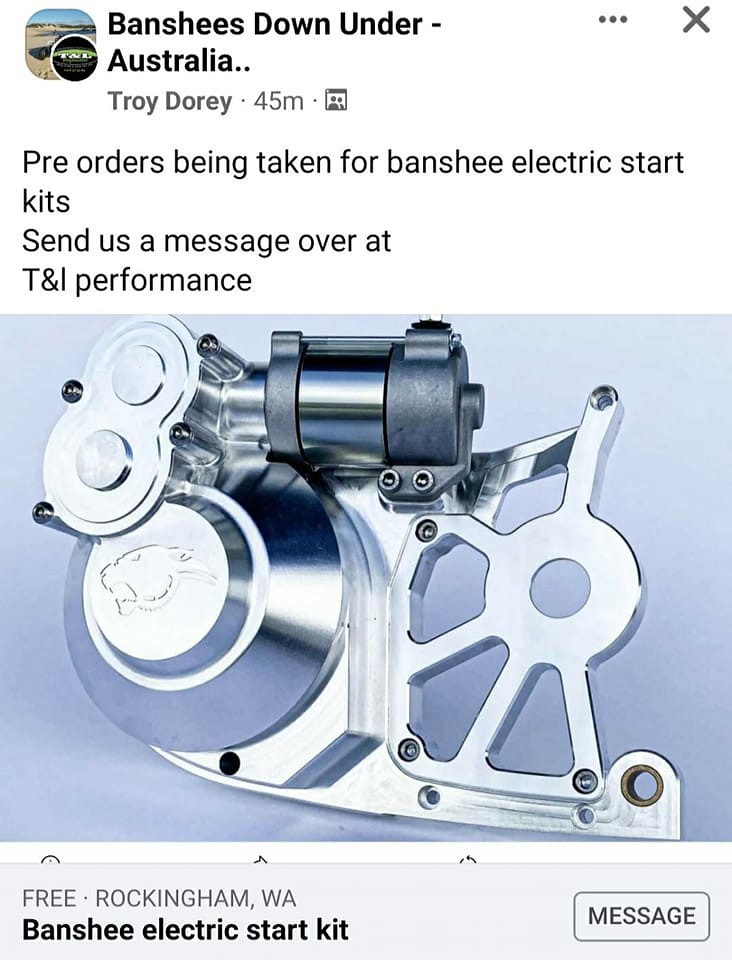The image is a screenshot of a Facebook post by "Banshees Down Under Australia," authored by Troy Dorey, posted 45 minutes ago. The post announces pre-orders for Banshee electric start kits and invites users to send a message to T&I Performance. The visual features a detailed image of the Banshee electric start kit, a shiny silver metallic assembly with a cylindrical black component on top. The kit consists of several metallic parts, some with circular holes, and a larger spinning spherical segment. A distinctive symbol resembling a saber-tooth tiger is visible on the left. Below the image, there's a grey banner indicating "Free Rockingham WA Banshee electric start kit" with a rectangular "MESSAGE" button on the right. An "X" symbol appears in the top right corner of the screenshot.